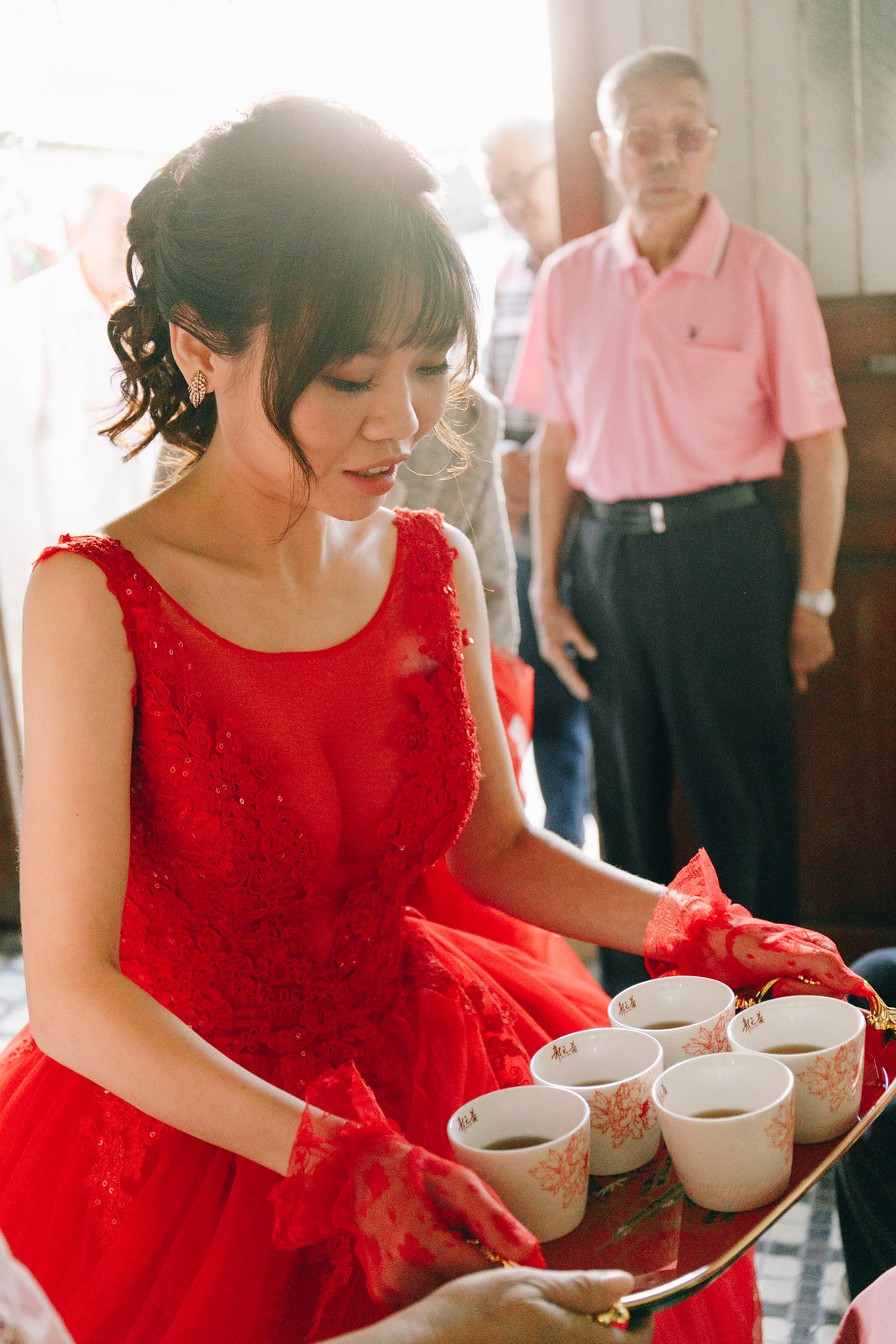In this detailed photograph of an indoor ceremony that feels somewhat like a wedding or a fancy get-together, a young Asian woman stands prominently in the foreground. She is elegantly dressed in a long, red lace dress that matches her red lace gloves. Her black hair is styled in an elaborate updo with bangs framing her face as she looks down at the tray she is holding with both hands. The tray holds five white mugs, each decorated with red floral accents, filled halfway with what appears to be tea.

In the background, various people are engaged in conversation. One man, who also appears to be Asian, stands out. He is older, with buzzed gray hair, and wears glasses. His outfit comprises a short-sleeved pink polo button-up shirt, long dark pants, and a belt. This man seems to be looking at the woman with the tray. The setting is illuminated by natural light streaming through a large doorway, further adding to the celebratory and somewhat formal atmosphere of the scene.